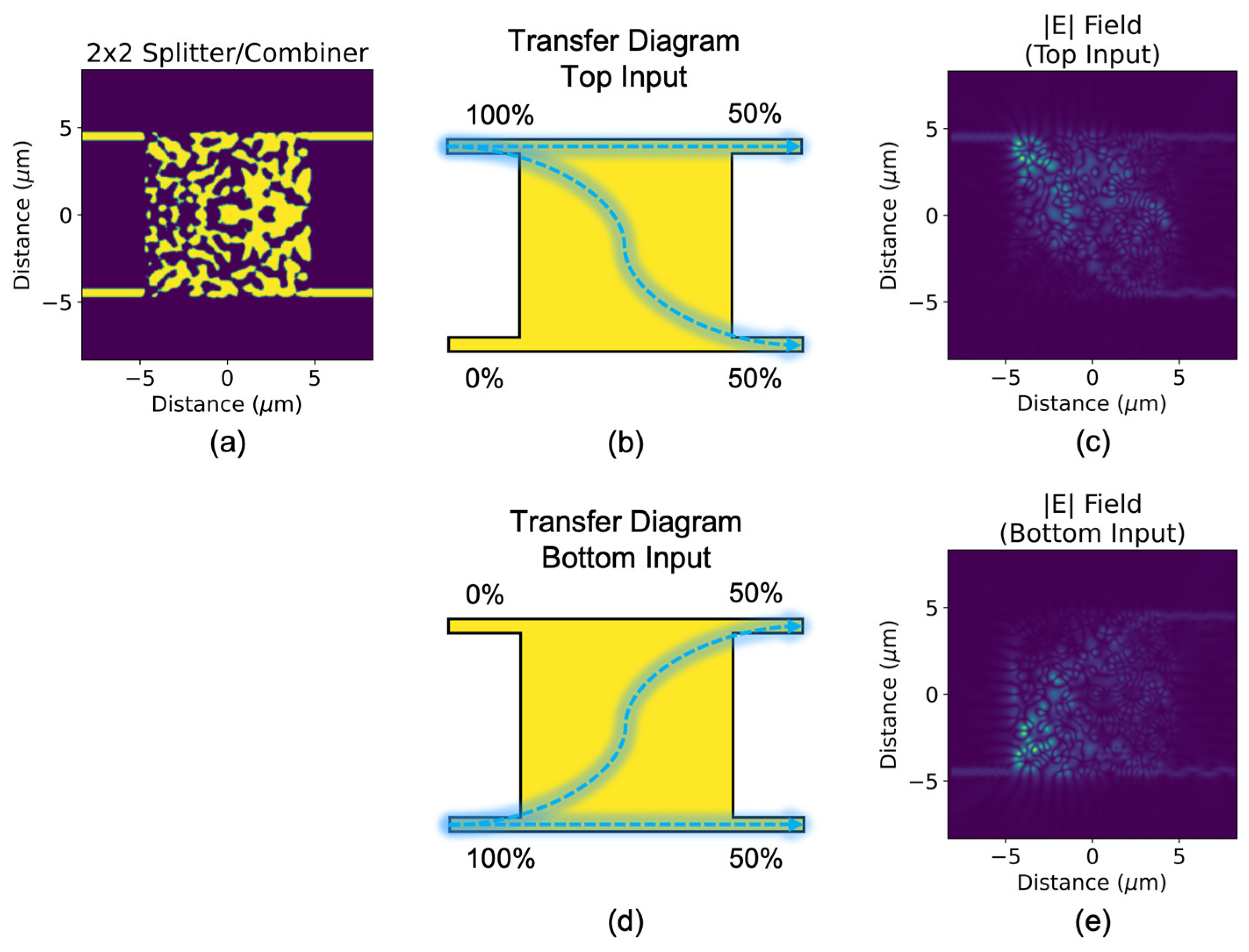The image contains a detailed scientific diagram set against a white background, featuring five distinct square images. In the top left, there's a dark purple square with yellow lines resembling a QR code. This image is titled "2x2 Splitter/Combiner" and contains X and Y axes labeled "Distance in Microns," ranging from -10 to 10 in increments of five. To its right near the upper corner is another dark purple square with faded spots of purple and green, titled "E Field Top Input," and it shares the same axes and scale as the first image. Directly below it, at the lower right, is a similarly designed square labeled "E Field Bottom Input."

In the center are two yellow squares with extended edges and dashed curved lines; both squares have a unique percent scale with one labeled "Transfer Diagram Top Input" and ranging from 0 to 50% on the bottom and 100% to 50% on the top. The other is a mirrored version labeled "Transfer Diagram Bottom Input," displaying 100% to 50% on the bottom and 0% to 50% on the top.

The axes, colors, and scales are consistent and aid in understanding the electric field and transfer data this diagram aims to convey, emphasizing a complex representation of scientific information potentially related to electrical measurements or field studies.